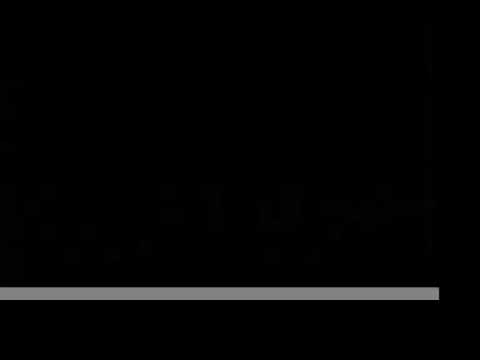This image features an entirely black background with a single, distinct gray line running horizontally near the bottom. The gray line spans almost the entire width of the image, but stops just short of the right edge, creating a small gap. The line is thin and uniformly flat on both the top and bottom sides. Positioned approximately one inch from the bottom edge, it lies within the bottom quarter to fifth of the image. The stark contrast of the gray line against the black background suggests a minimalist, preliminary stage of a digital or artistic creation. There are no other objects, text, or colors present in the image.